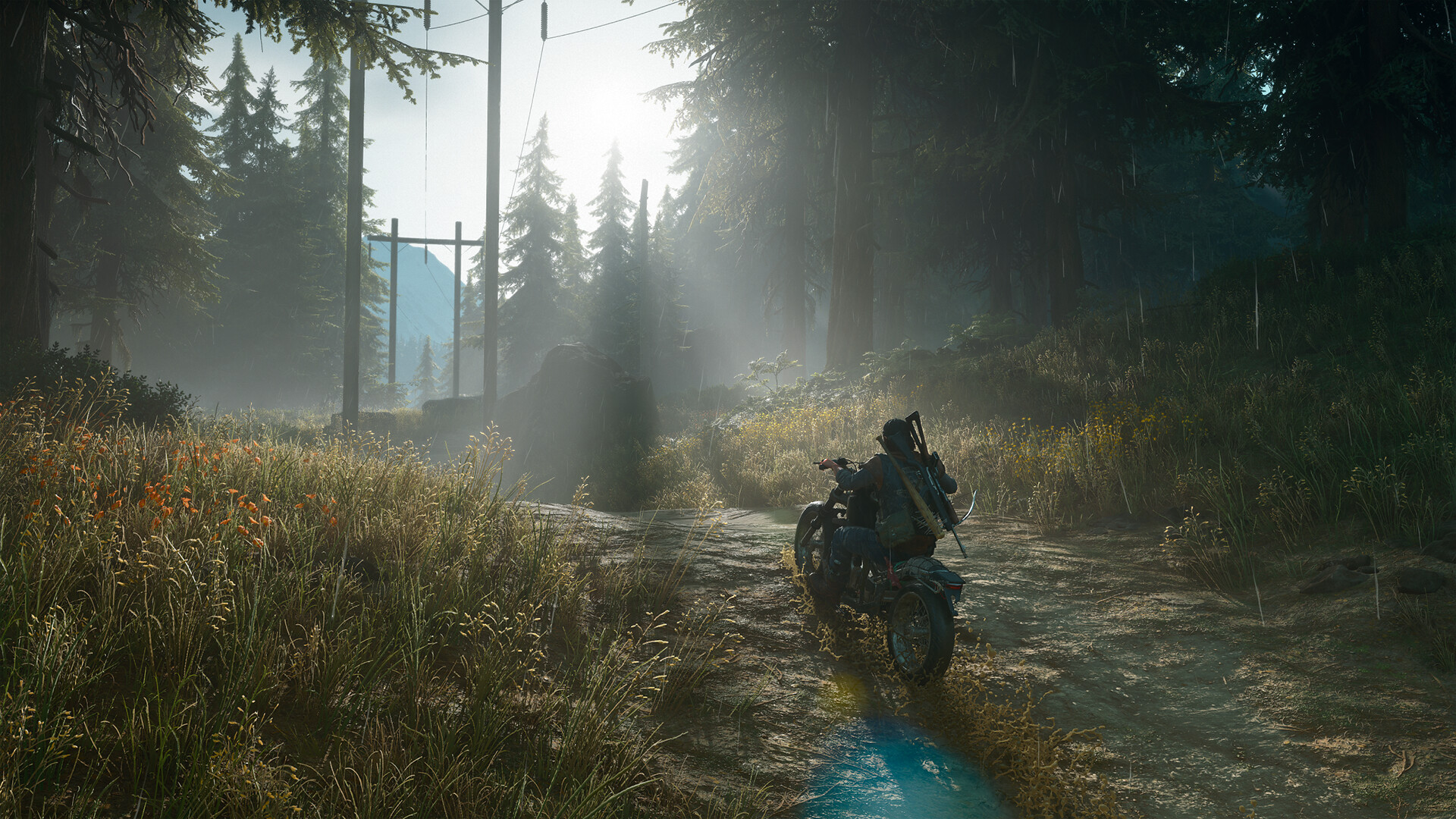A dirt trail winds through a dense forest of dark green evergreens, leading into the distance towards a mountaintop, under an array of power lines held up by imposing pylons. The scene, which appears hyper-realistic or like a meticulously detailed AI-generated image, features a person on an old-fashioned motorcycle from the 50s or 60s. They are shaded and facing away from us, positioned slightly right of center on the trail. The motorcycle has just crossed a small blue puddle. The rider wears a gray jacket, long pants, and carries a bat and a rifle on their back. The light filters down from the sky, creating rays above the pine trees that line both sides of the trail. Besides the dark evergreens, the trail is bordered by green grasses and various wildflowers. This picturesque, almost surreal image captures a moment of solitary adventure amidst nature's bounty.